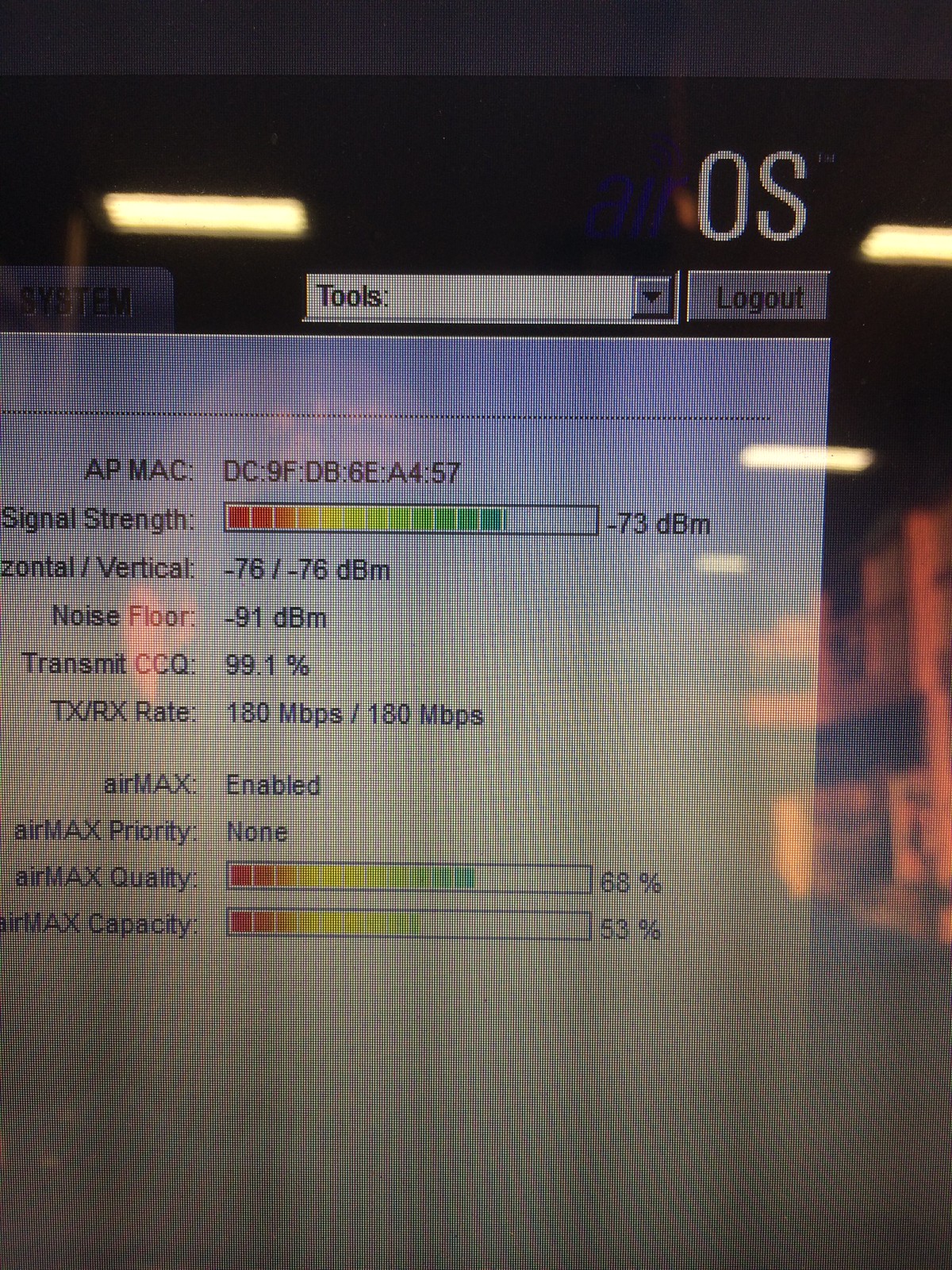The image captures a close-up of a computer monitor displaying a detailed page of information, seemingly part of a software interface related to network statistics or performance metrics. The screen has noticeable scan lines typical of photographs taken of monitors, adding a textured, grid-like pattern overlay. Reflections on the screen suggest it was taken by someone wearing a cap, and ambient lights are visible in the background.

In the upper right corner of the white page, the text "OS" is displayed against a black header. Just below it is a tools dropdown menu and a "Log out" button to the right. Central to the screen is the main content area, listing various metrics: 

- "AP Mac" with a code: "DC 9FDB6EA457"
- "Signal strength," shown with a color-coded bar from red to green indicating a value around -73 dBm
- "Horizontal / Vertical" listed as -76 / -76
- "Noise floor" at -91 dBm
- "Transmit CCQ" at 99.1%
- "TX RX rate" indicating 180 Mbps / 100 Mbps

Further down, "Air Max" features are outlined:

- "Air Max" status: Enabled
- "Air Max priority": None
- "Air Max quality," illustrated with another red-yellow-green bar, achieving 68%
- "Air Max capacity," also displayed with the colored bar, reaching 53%

Bordering this detailed display, the crisscross patterns of lines hint at some interference from capturing the image through a screen or fence-like structure, adding an abstract element to the technical content.